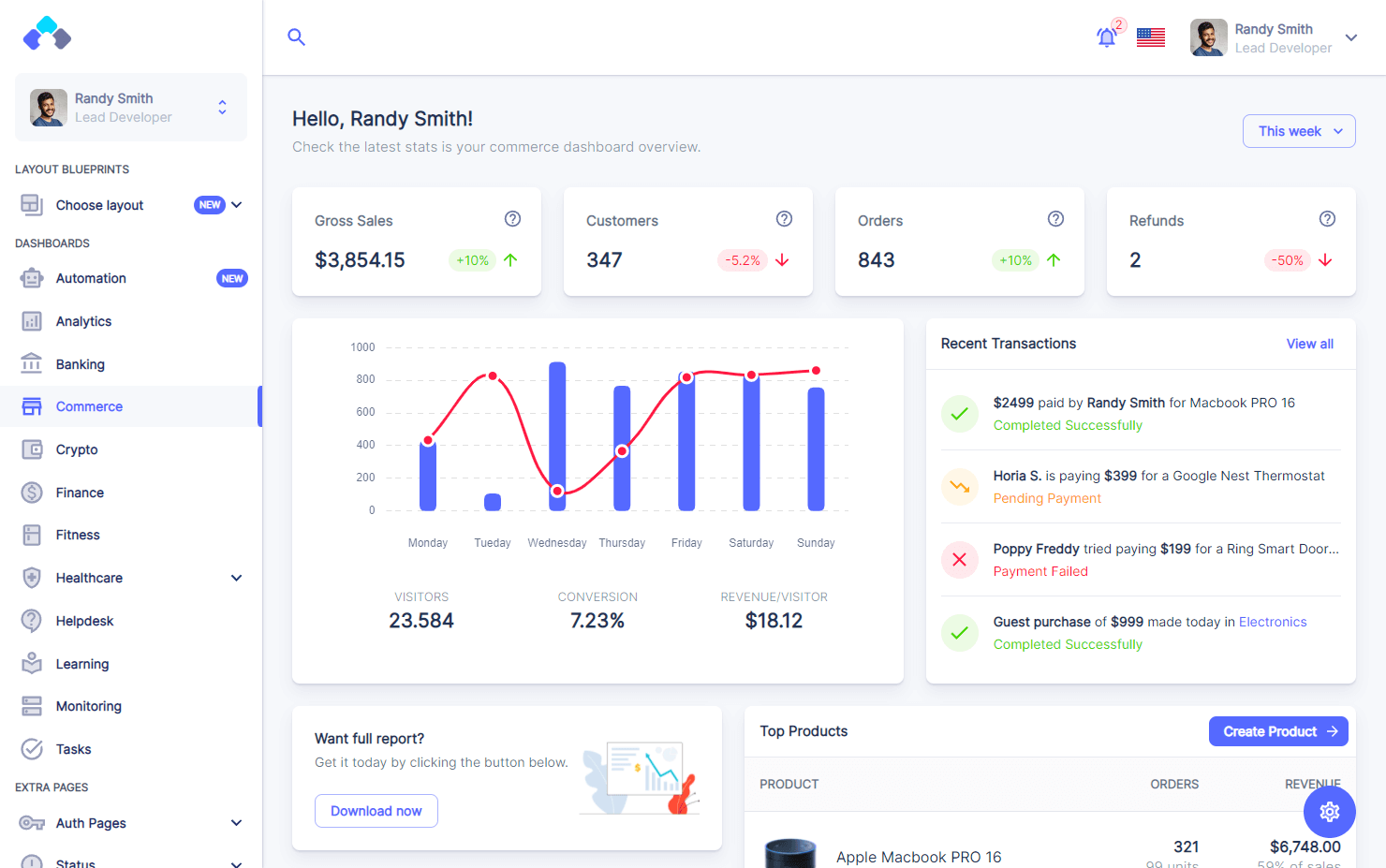**Detailed Caption:**

In the top right corner of the dashboard, there is a notification bell icon followed by the number 2, indicating two new notifications. Adjacent to this is an American flag icon representing localization settings. Below these icons, the text "Randy Smith, Lead Developer" is prominently displayed. 

The top left corner of the dashboard features a blue-themed icon. Along the left-hand side of the layout, there is a side navigation panel with various categories labeled "Layout Blueprints," "Dashboards," "Automation," "Analytics," "Banking," "Commerce," "Crypto," "Finance," "Fitness," "Healthcare," "Helpdesk," "Learning," "Monitoring," "Tasks," and "Extra Pages." Each category is accompanied by respective icons, such as a robot head for automation, a graph for analytics, and a shopping cart for commerce.

Midway on the dashboard, there is an option to "Choose Layout," displayed as a blue oval button with the label "New." Just below this, in the main view area of the dashboard, is the text "Hello Randy Smith, check the latest stats. This is your commerce dashboard overview."

The weekly summary includes:
- *Gross Sales:* $3,854.15, with an approximate 10% increase.
- *Cost:* 0.2%, contributing to a total of 95.2%.
- *Real Estate Investments:* $430, with a change of plus 2 and a decrease of 50%.

The dashboard graphically represents the flow of visitors from Monday to Sunday. The section for recent investments highlights a total of $2,049.00, including a payment of $3.99 to Google, accounting for 2%. Additionally, Randy Smith has recently purchased a MacBook Pro 16 for himself.

Overall, this dashboard provides a comprehensive overview of the latest commerce-related statistics and recent transactions efficiently and effectively.